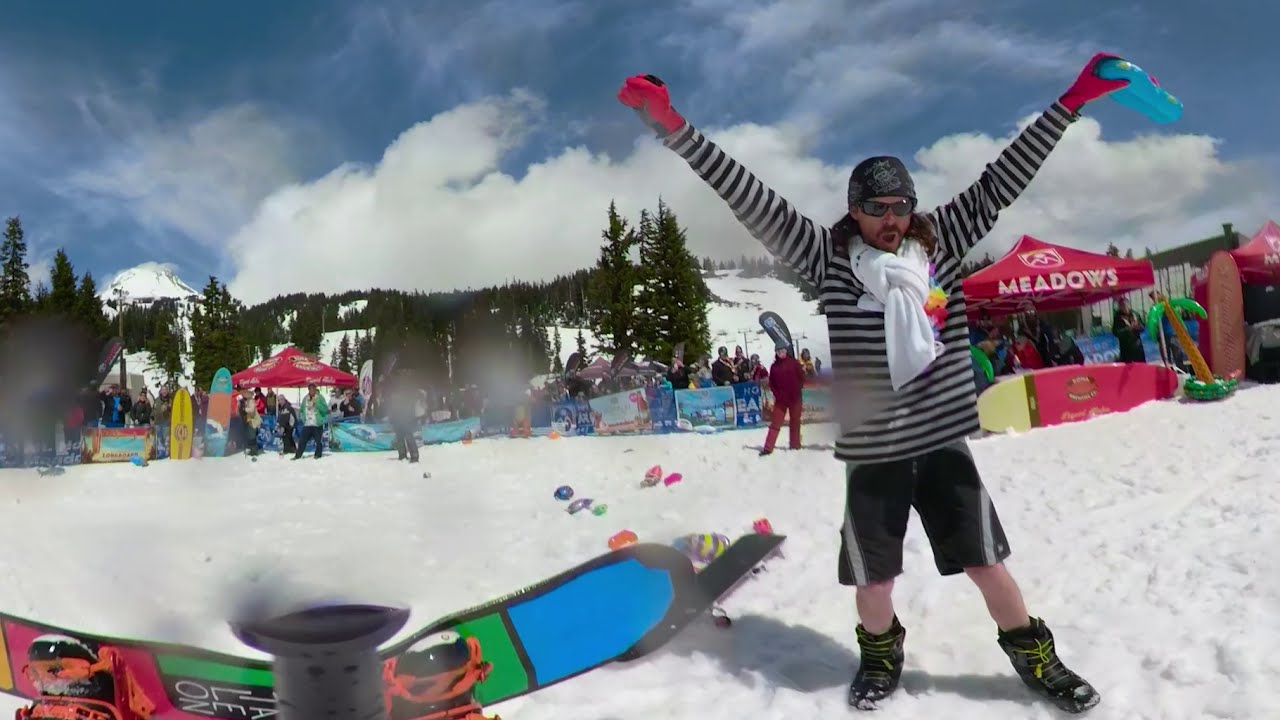In this outdoor, snow-covered scene set in the middle of the day, a triumphant man stands slightly to the right of center, raising his arms in victory. He is dressed in a black and white horizontally striped shirt and black shorts with vertical silvery stripes, complemented by red gloves, a white scarf, goggles, a cap, and black shoes with fluorescent yellow-green laces. In his left hand, he holds a blue object. 

Surrounding him, the ground is blanketed with snow. To his right, a multicolored snowboard in shades of blue, green, red, and orange lies in the snow. A red and yellow tent with the word "Meadows" printed on it is visible under his left arm, likely a vendor's tent. The background features a hillside or mountainscape view adorned with pine trees, various canopies, snowboards standing up, and people dressed for the cold weather. Notable figures include a person in green, white, and blue attire, and another in a reddish outfit. The sky above is mostly covered in clouds, casting a light gray tone over the scene. This vibrant image is awash with several colors including blue, gray, white, green, red, light blue, yellow, orange, purple, and pink, reflecting a lively and dynamic outdoor event.